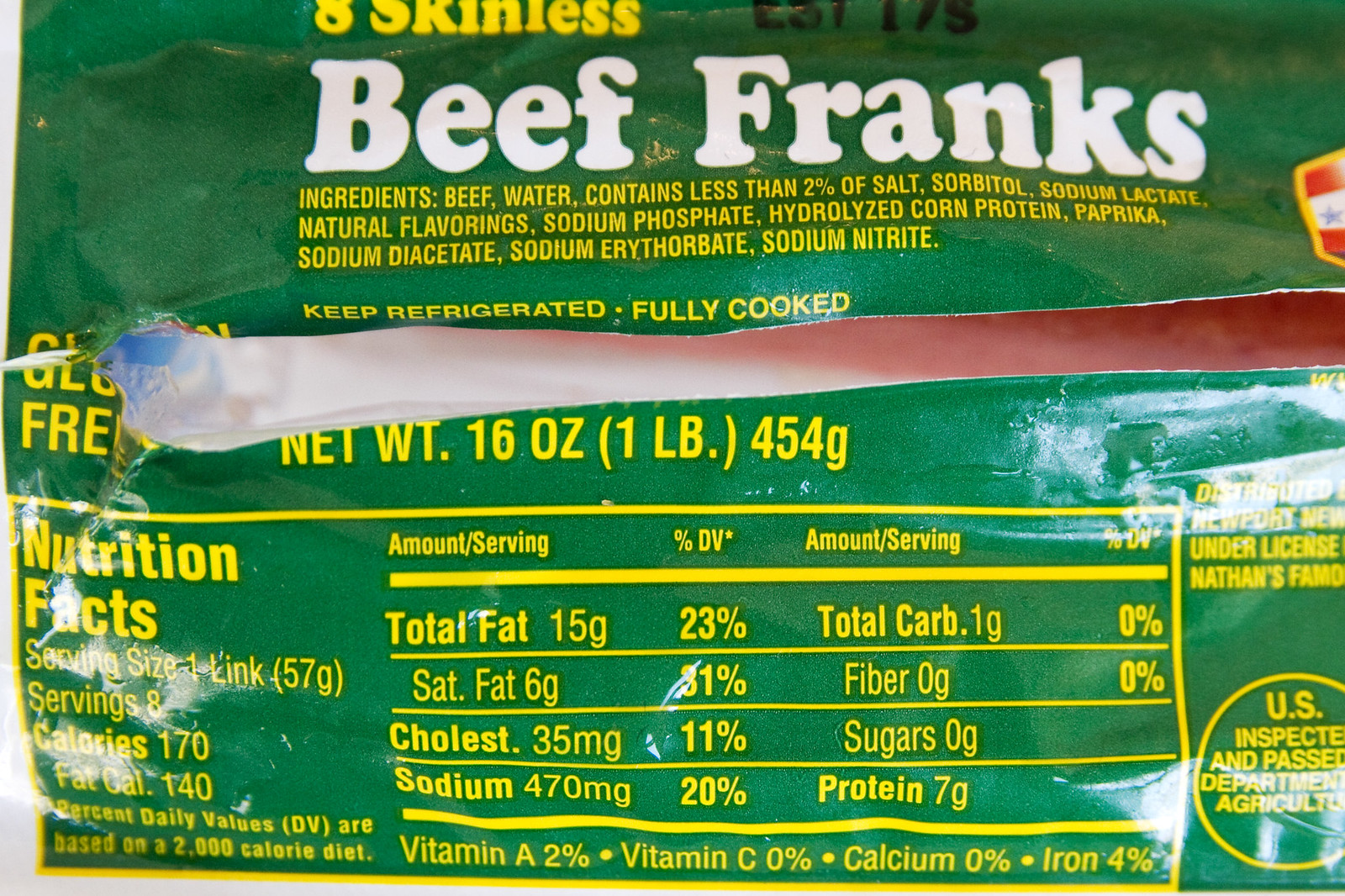The image is a horizontally rectangular photograph of an open package of hot dogs, set against a medium, grass-green background. The package, viewed from a lateral perspective, features prominently in the frame and has a slit going from left to right. The hot dog package is primarily green with yellow and white writing. At the top, it prominently states "Eight Skinless Beef Franks" in white text. Below this, in yellow, are directives such as "Keep Refrigerated" and a clarification that the hot dogs are "Fully Cooked."

On the left side of the packaging, partly obscured by the tear, it mentions "Gluten-Free." The package's net weight is 16 ounces or 1 pound (454 grams). The nutrition facts below this indicate that each serving is one link, with the package containing eight servings. Each serving has 170 calories, of which 140 are from fat. Detailed nutritional information reveals 15 grams of total fat (23% DV), 6 grams of saturated fat (31% DV), 35 milligrams of cholesterol (11% DV), 470 milligrams of sodium (20% DV), 1 gram of total carbohydrates (0% DV) with no dietary fiber or sugars, and 6 grams of protein. The lower right corner of the package displays an inspection seal from the U.S. Department of Agriculture. Ingredients listed include beef, water, and less than 2% of various additives like salt and paprika.